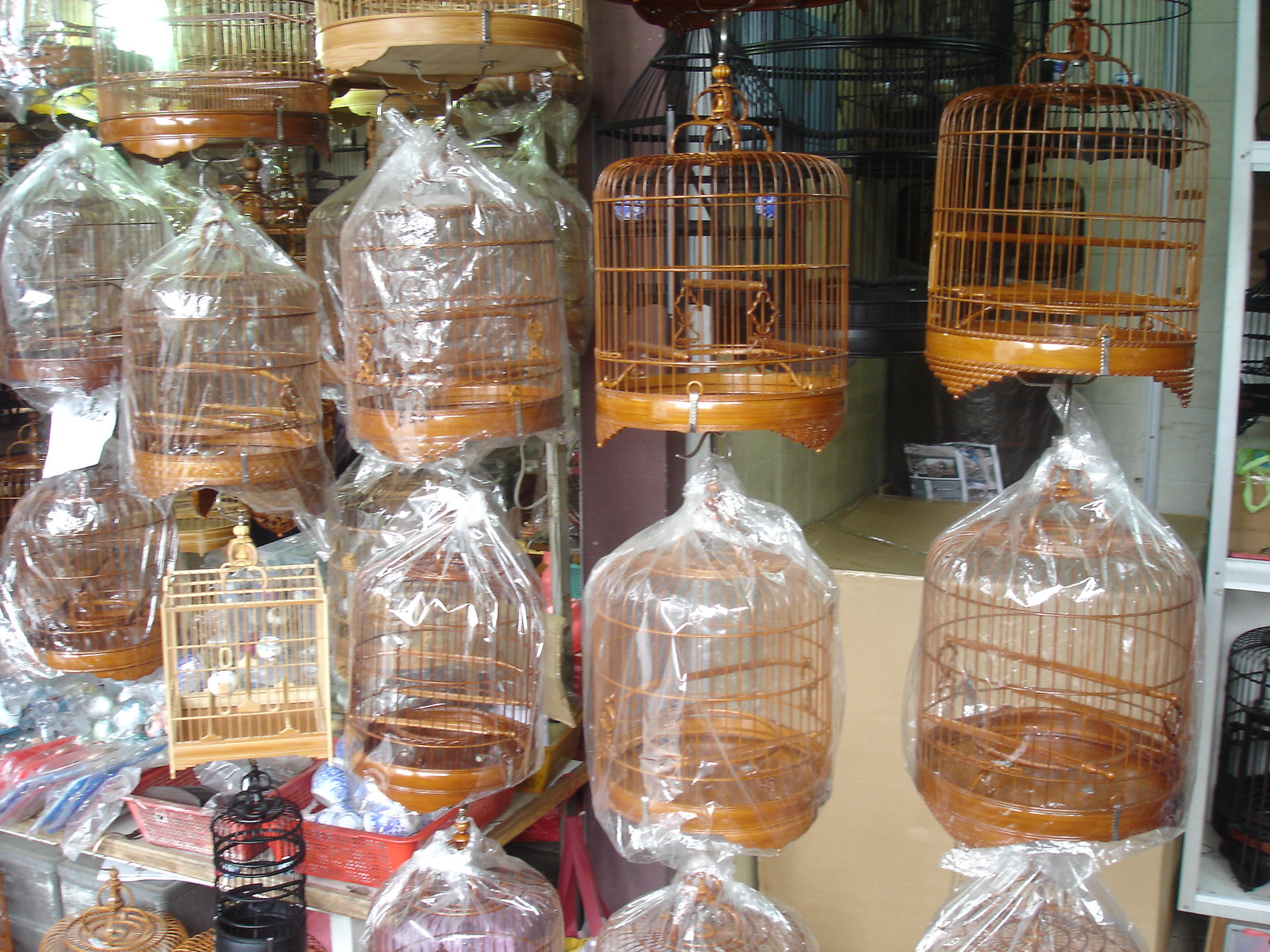The image displays an assortment of bird cages artistically suspended from the ceiling. The primary cages are uniform in a metal brown, brass-like color, and cylindrical with rounded tops, each featuring a hook for hanging. These cages are interconnected, with some hanging from others, creating a cascading effect. In clear view, there are approximately 15 to 16 bird cages, most wrapped in transparent plastic except for a few—specifically four to six—that remain uncovered. A prominent, pale square bird cage can be seen slightly to the left amidst the predominantly round cages. 

The background reveals additional details: behind the right row of cages, a closed cardboard box sits, flanked by a tall white shelving unit with at least three visible shelves, extending upward beyond the frame. To the left, a collection of plastic bags and a red crate are noticeable beneath the hanging cages. The setup hints at a storefront environment, with the bird cages displayed above a table featuring red trays containing various items, alongside more cages partially visible in a bookcase-like arrangement to the far right.